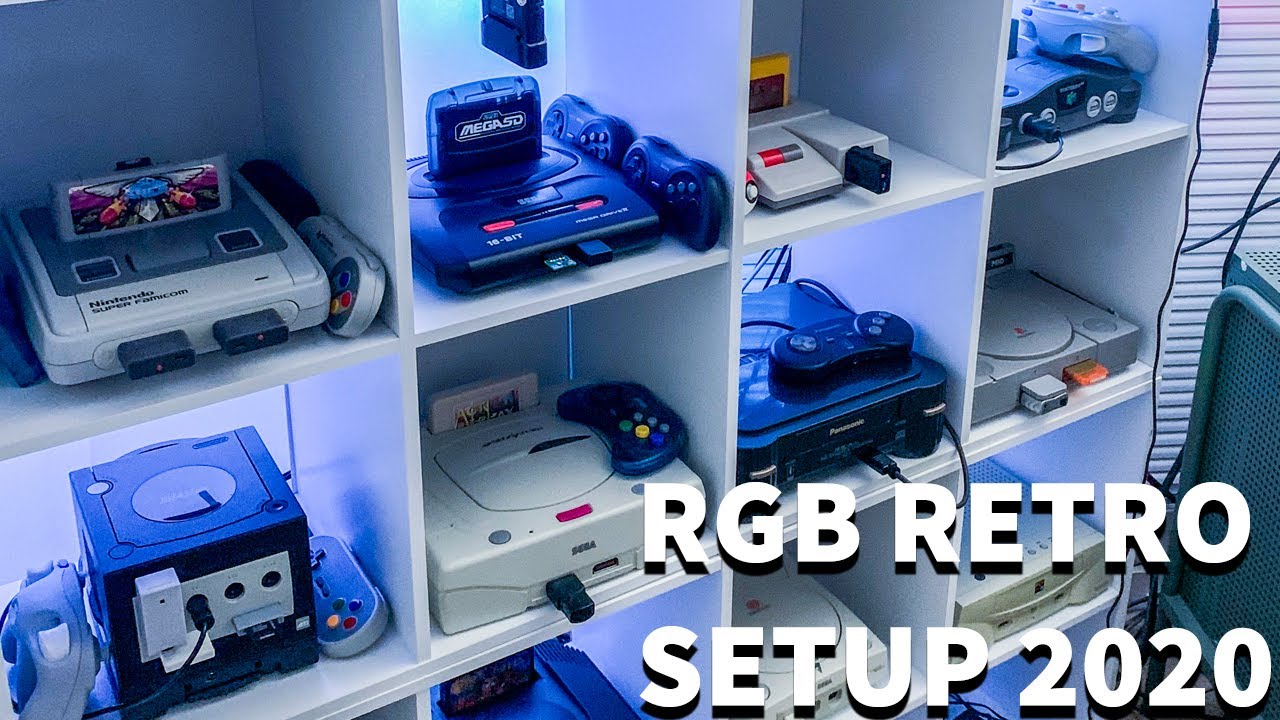This photograph showcases a close-up view of a large shelving unit, likely resembling an IKEA Lack shelf, filled with an array of retro gaming consoles and their respective controllers. The unit is captured from a slightly left-facing angle, hinting at more compartments than visible. The visible section comprises 11 cubby holes arranged in four columns and at least three rows, although the actual structure may contain additional rows and columns extending beyond the frame.

Each cubby hole is home to a classic gaming system. In the top row from left to right, the visible consoles include a Nintendo Super Famicom (the Japanese version of the Super Nintendo), a Sega Mega Drive, an unidentified console, and a Nintendo 64. The second row features a Nintendo GameCube on the left, followed by another Sega console, a Panasonic device, and a PlayStation 1. The third row, only partially visible, contains what appears to be another Sega console and an unidentified system.

Adding a modern touch to this nostalgic display, the bottom right corner of the image is inscribed with the phrase "RGB Retro Setup 2020," suggesting the photograph may have been taken for a blog or social media showcasing the owner’s retro gaming collection. Adjacent to the shelving unit, a green object, possibly a chair, is partly visible. This visually rich setup pays homage to the golden era of video gaming, meticulously organized within this multi-cubby shelving unit.